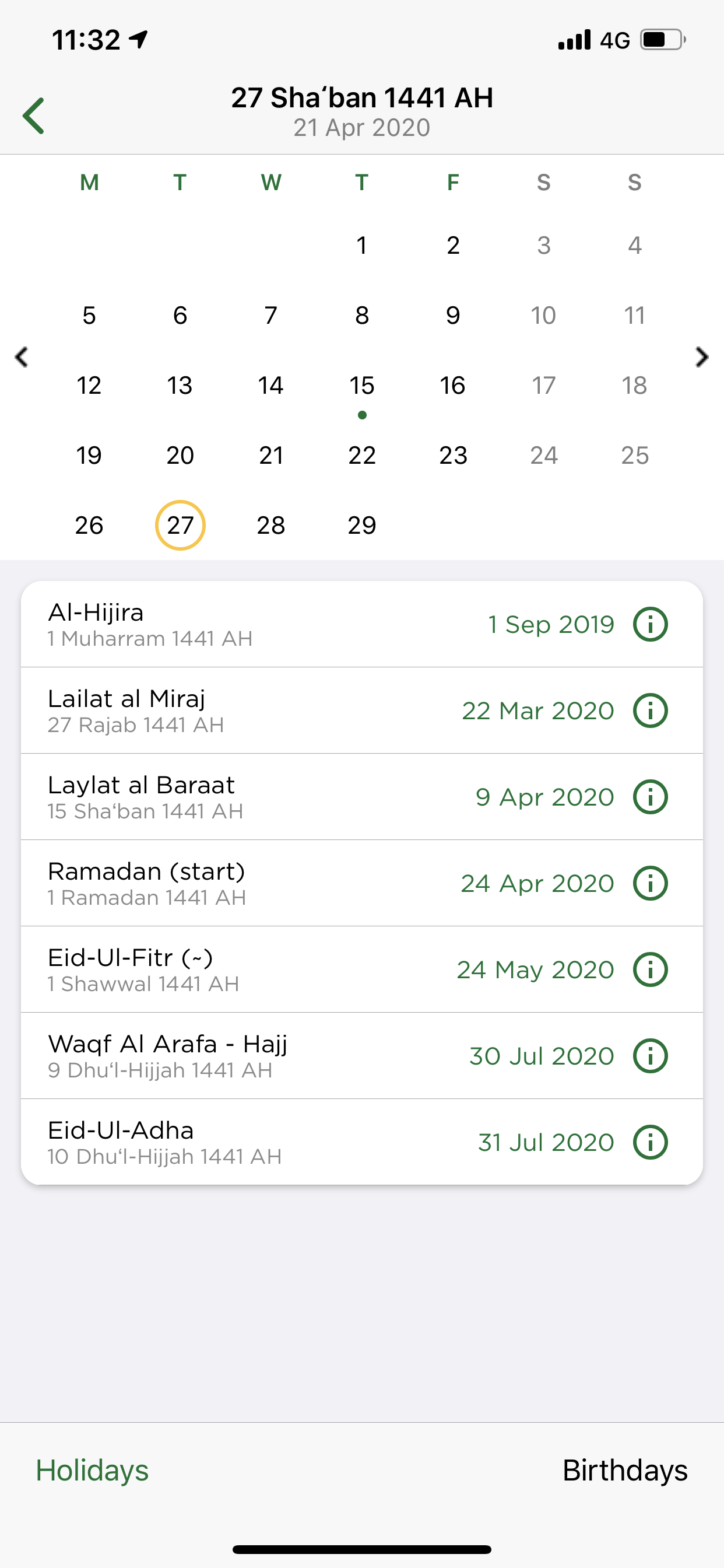A clean and descriptive caption:

"This is a detailed screenshot of a calendar app on a smartphone, captured at 11:32 AM with a 50% battery level and a 4G connection. The background is a subtle off-white. At the top of the app, the date reads '27 Shaban, 1441 AH, 21 April 2020.' Directly below this header is the calendar for April 2020.

The calendar layout shows that the month begins on Thursday, April 1st, and ends on Thursday, April 29th. Notably, Tuesday, April 27th, is circled in yellow, indicating a significant date. Additionally, there is a green dot beneath Thursday, April 15th. Below the calendar, several entries are listed: 'Al Ajari, 1 September 2019,' 'Lailat Al Miraj, 22 March 2020.'

At the very bottom of the screenshot, two tabs are visible: on the left, 'Holidays,' and on the right, 'Birthdays,' allowing the user to toggle between different calendar views."